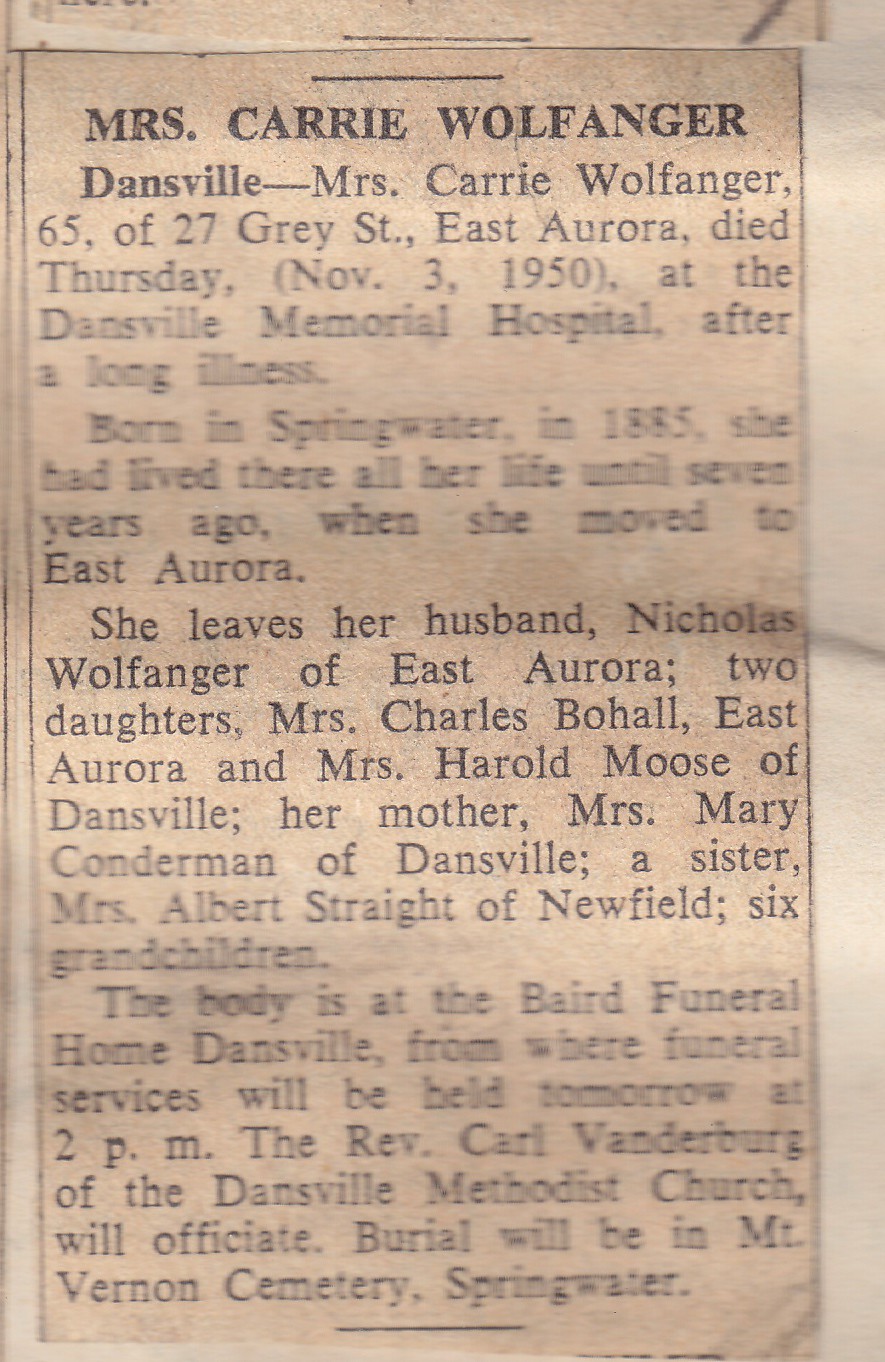The image is of a yellowed and aged obituary from a newspaper, dated November 3, 1950. The headline, "Mrs. Carrie Wolfanger, Dansville," is prominently printed in bold black lettering. Mrs. Carrie Wolfanger, aged 65, who resided at 27 Gray Street, East Aurora, passed away at the Dansville Memorial Hospital after a prolonged illness. Born in Springwater in September 1885, she spent most of her life there before relocating to East Aurora seven years prior to her death. She is survived by her husband Nicholas Wolfanger of East Aurora, two daughters, Mrs. Charles Bohol of East Aurora, and Mrs. Harold Moose of Dansville, as well as her mother, Mrs. Mary Konderman of Dansville. Also mourning her loss are her sister, Mrs. Albert Strait of Newfield, and six grandchildren. Funeral services are to be held at Baird Funeral Home in Dansville at 2 p.m. the following day, officiated by Reverend Carl Vandenberg of the Dansville Methodist Church. Interment will take place at Mount Vernon Cemetery in Springwater. The obituary article is noticeably worn, with the paper taking on a light brown hue over time.